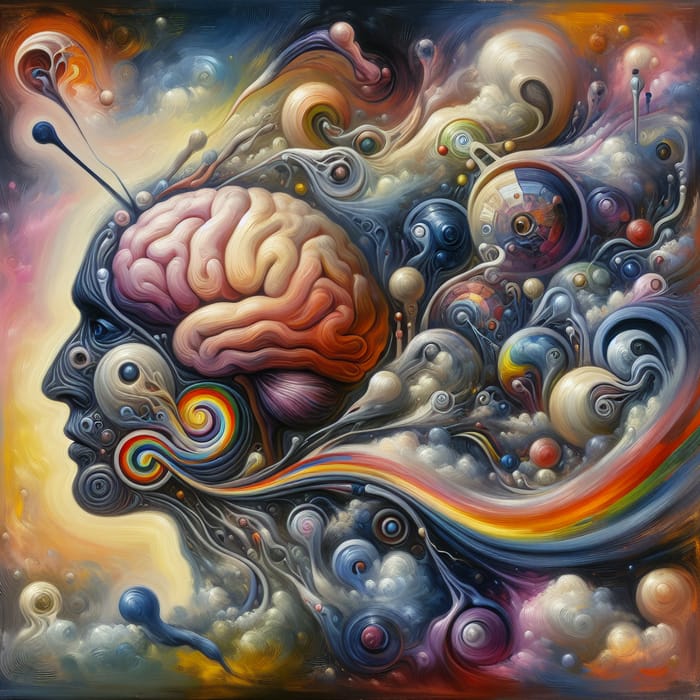The image is a square, psychedelic-style painting with no border or definitive background, predominantly featuring the side profile of a humanoid head located in the center-left. The face, depicted in shades of blue with various intricate swirls, prominently displays an exposed brain rendered in purple, white, and orange hues. Above the brain and surrounding the head are rainbow-colored ribbons twisting and spiraling outward, creating a dynamic, flowing effect across the image. The cheek of the face contains swirls that blend into the rainbow ribbons, which shoot off to the right, forming artsy circles composed of reds, oranges, yellows, greens, blues, and purples. Both lower corners of the painting showcase wispy clouds, contributing to the celestial, dreamlike atmosphere. Additional geometric shapes can be seen in the upper left-hand corner, enhancing the abstract, new-agey aesthetic.